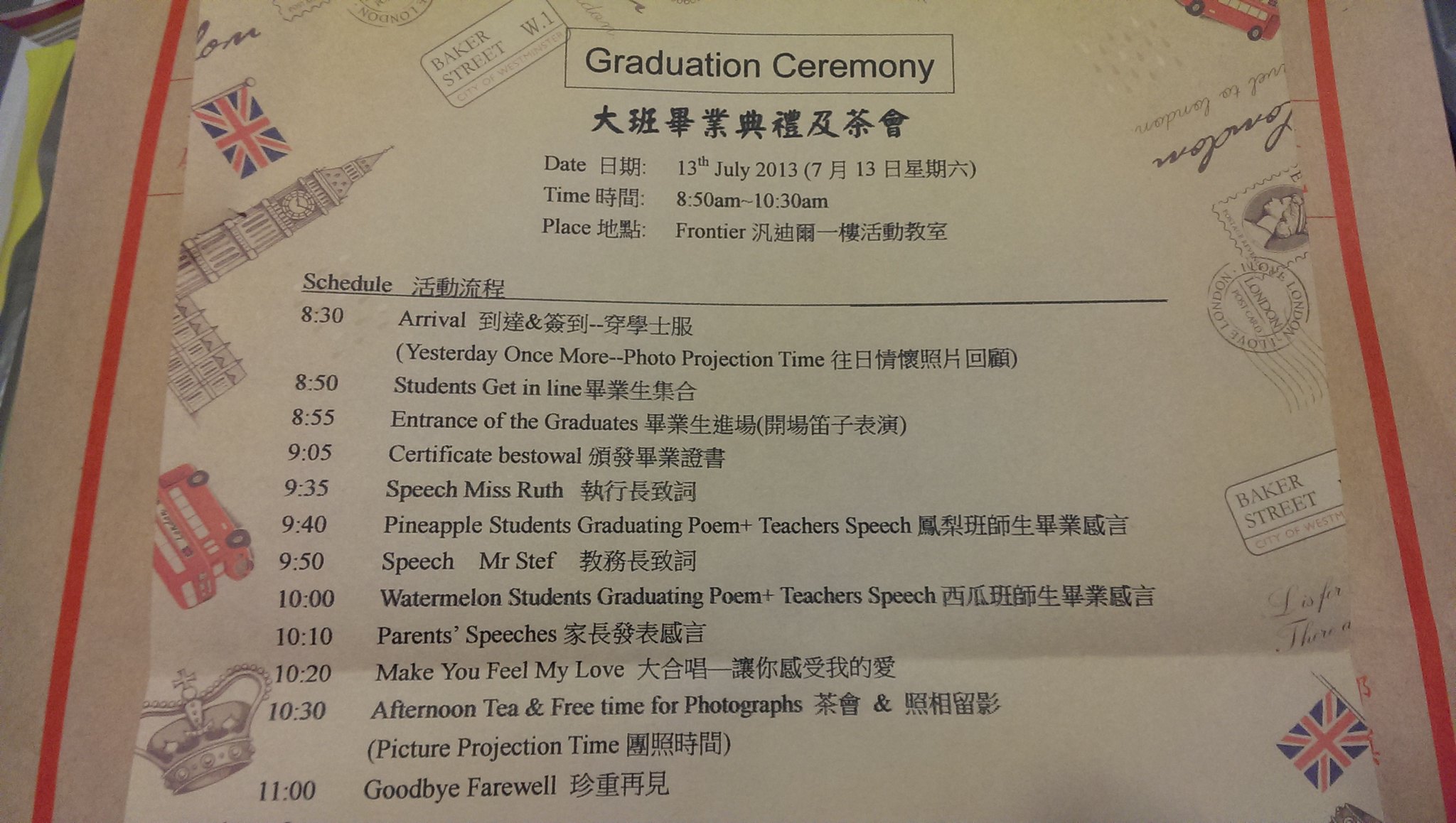This photograph captures a detailed graduation ceremony schedule printed on an elaborately themed piece of paper. The schedule is for a ceremony held on July 13th, 2013, from 8:50 a.m. to 10:30 a.m. at a place called Frontier. The design of the paper is particularly striking, featuring iconic British symbols such as Big Ben, the Union Jack, red double-decker tour buses, and Baker Street along its edges.

The top of the schedule is titled "Graduation Ceremony," followed by text in Chinese characters. Below this header, the schedule outlines events starting at 8:30 a.m. with arrival, 8:50 a.m. for students getting in line, and 8:55 a.m. for the entrance of graduates. The ceremony continues with the bestowal of certificates at 9:05 a.m., a speech by Miss Ruth at 9:35 a.m., followed by a graduation poem and a teacher's speech by the Pineapple Students. The morning concludes with the song "Make You Feel My Love," afternoon tea, and free time for photographs, culminating with a farewell at 11:00 a.m. The schedule is presented in English, accompanied by Chinese characters, reflecting a bilingual arrangement.